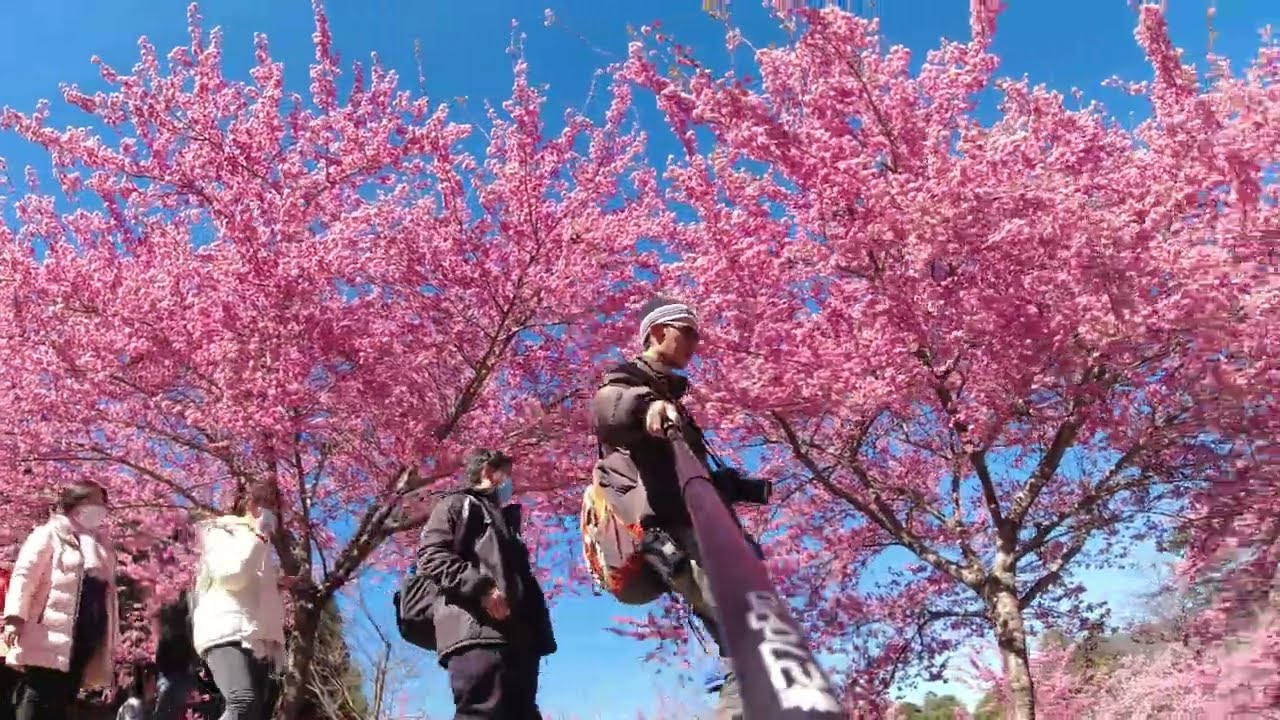This captivating photograph, likely taken during a cherry blossom festival, provides a unique perspective from a selfie stick held towards the ground by the photographer at the front of a line of four people. The image captures vibrant pink cherry blossoms in full bloom, contrasting against a bright, perfectly blue sky with a few clouds hovering over a hillside in the bottom left corner. The hillside features some plants and small trees growing from its mainly dirt surface.

The person taking the selfie is wearing a gray beanie, sunglasses, and a black backpack, and is dressed in a black jacket. He is the only one not wearing a face mask, unlike the other three individuals behind him. The second person, a man in all black with a backpack and face mask, is followed by two women in lighter-colored jackets but dark pants, who are also wearing face masks. The selfie stick has some numbering and Chinese letters visible on it. The angle from which the photograph is taken offers a dynamic view, emphasizing the rich pink blossoms against the tranquil blue sky, making it a truly captivating shot.